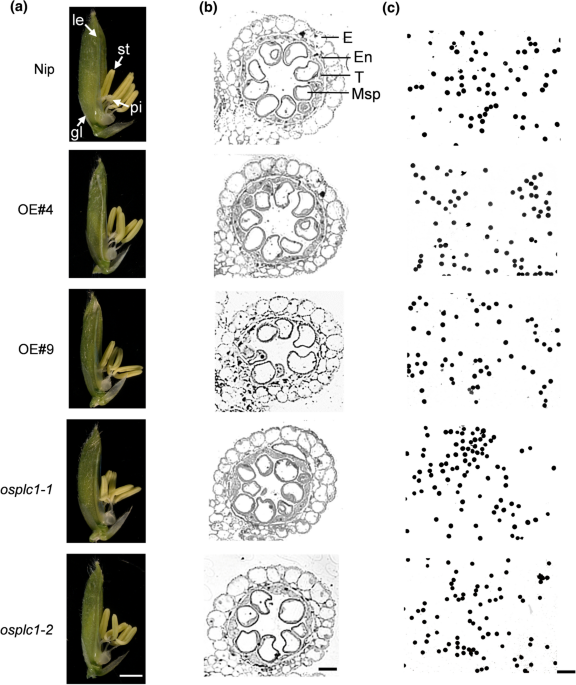The image is a detailed scientific chart in portrait orientation, focusing on the analysis of a plant, likely detailing stages of its reproductive parts. The chart is organized into three vertical columns labeled (A), (B), and (C), with five rows corresponding to different developmental stages or conditions, labeled NIP, OE4, OE9, OSPIC 1-1, and OSPIC 1-2.

Column (A) on the left features five color photographs, each showing a green bud with yellow stamens and several pistils protruding from the base. The photographs seem to document slight variations in the positioning of the stamens across different stages or conditions.

Column (B) in the center contains black line art illustrations that correspond to the activities depicted in the photographs to the left. These diagrams are labeled with letters E, EN, T, and MSP, indicating different parts or sections of the plant's reproductive system.

Column (C) on the right displays scatter plots with black dots representing some form of density or distribution related to the illustrations and photographs in columns A and B.

This infographic blends photographic images, scientific drawings, and analytical charts to provide a comprehensive botanical informational chart, showcasing the detailed stages of plant development and reproductive physiology.